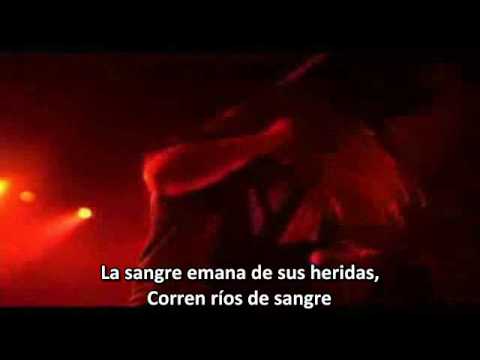The image features a predominantly black background swirled with intense splashes of red and orange hues. To the left, there are a couple of yellow light beams cutting through the vivid red area, creating bright circles which diffuse lighter reds and oranges, reminiscent of lights shining through a thick, reddish mist. The foreground and much of the image are blurred, making it difficult to discern specific objects but adding to the abstract and fiery appearance. Across the lower portion of the image, striking white text in Spanish reads, "La sangre emana de sus heridas, corren ríos de sangre," translating to "The blood emanates from his wounds, rivers of blood flow." The white text starkly contrasts against the dark, vibrant background, drawing the viewer's attention and likely serving as the focal point of the composition.